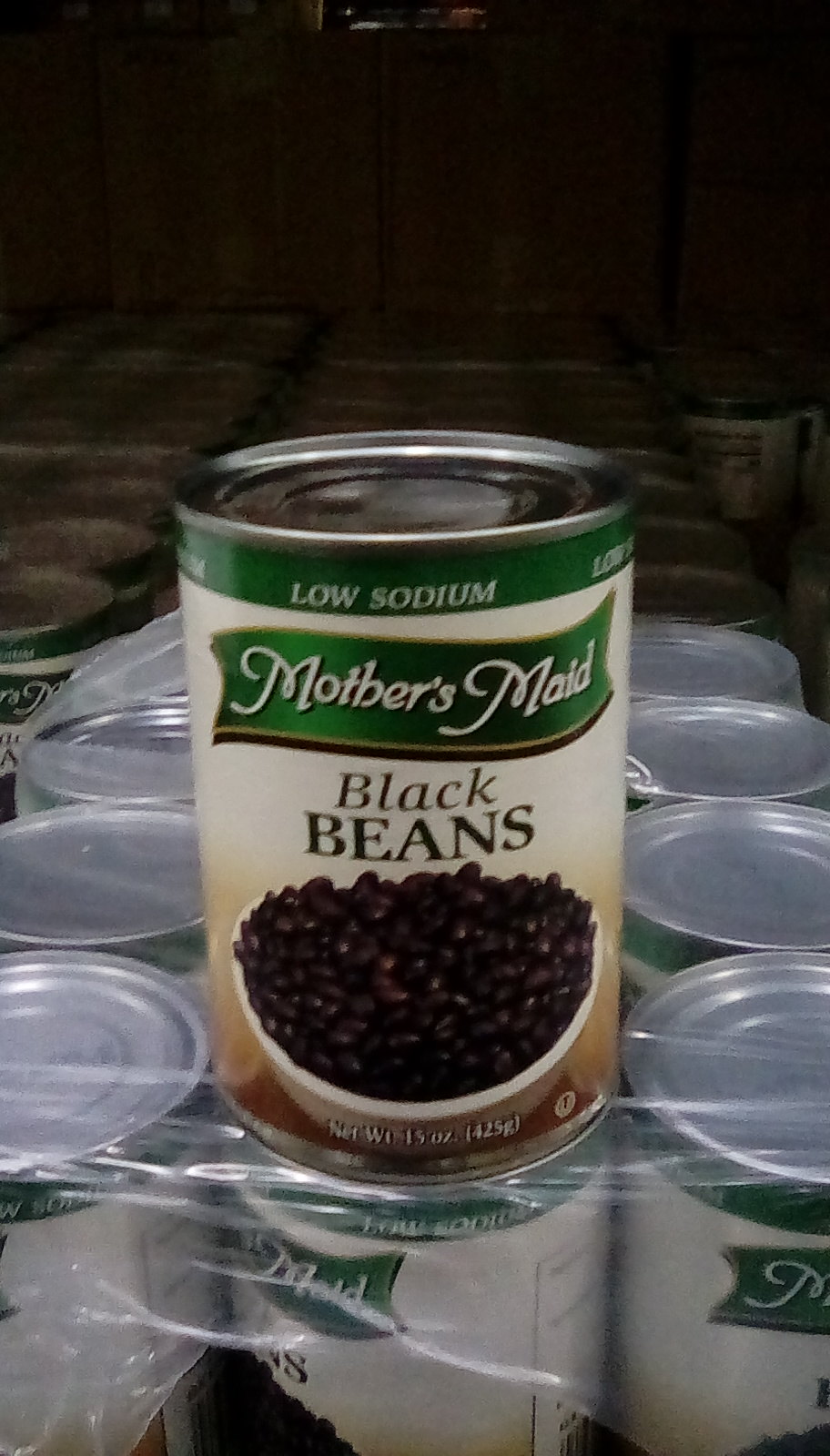This photograph is a close-up taken on a grocery store shelf, focusing on a prominently displayed can of Mother's Maid Low Sodium Black Beans. The can, featuring a green ribbon at the top with "Low Sodium" inscribed in white letters, rests atop a plastic-wrapped case of black beans, arranged in three rows of four cans each. The label is mostly white, accented with a green banner that reads "Mother's Maid" in white text, followed by "Black Beans" in larger black letters. Below this text, an image of a simple white bowl brimming with black beans is prominently displayed. The can's lid is silver, and the overall net weight is listed at 15 ounces. The background is dark and not well lit, but the shelved rows of plastic-wrapped cans extend into the distance up to a dark wall.